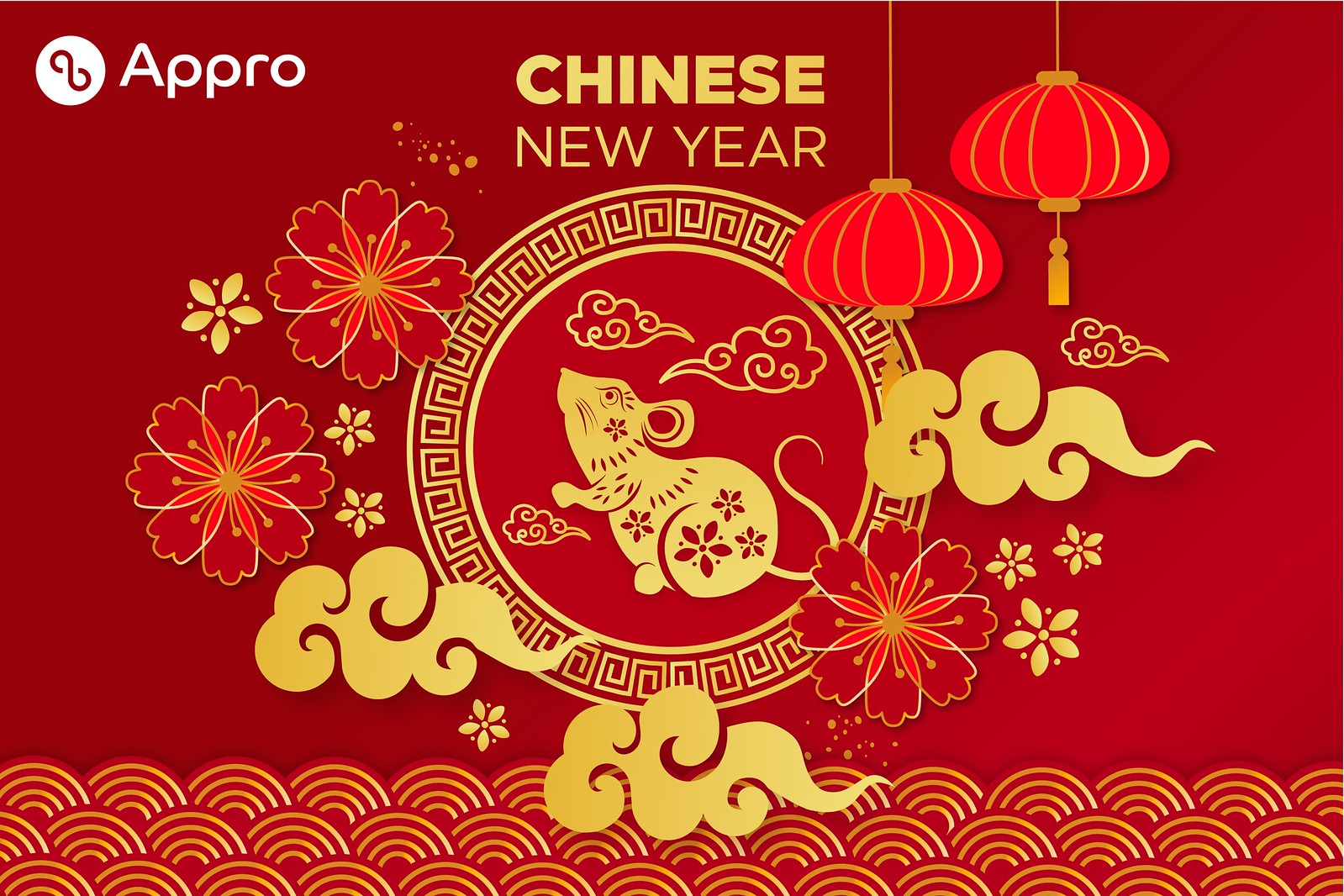The image features a vibrant red background with intricate details in gold and light red. At the center, there is a beautifully designed golden rat adorned with a floral pattern, symbolizing Chinese New Year. Surrounding the rat, there are decorative elements including yellow and red flowers, lotus flowers, and red Chinese lanterns. The design is also embellished with swirling clouds and wavy circular patterns at the bottom. In the top left corner, the words "App Pro" appear in white with an adjoining half-infinity symbol, while "Chinese New Year" is prominently written in the top middle of the image. The combination of these elements creates a rich and festive representation for the celebration.